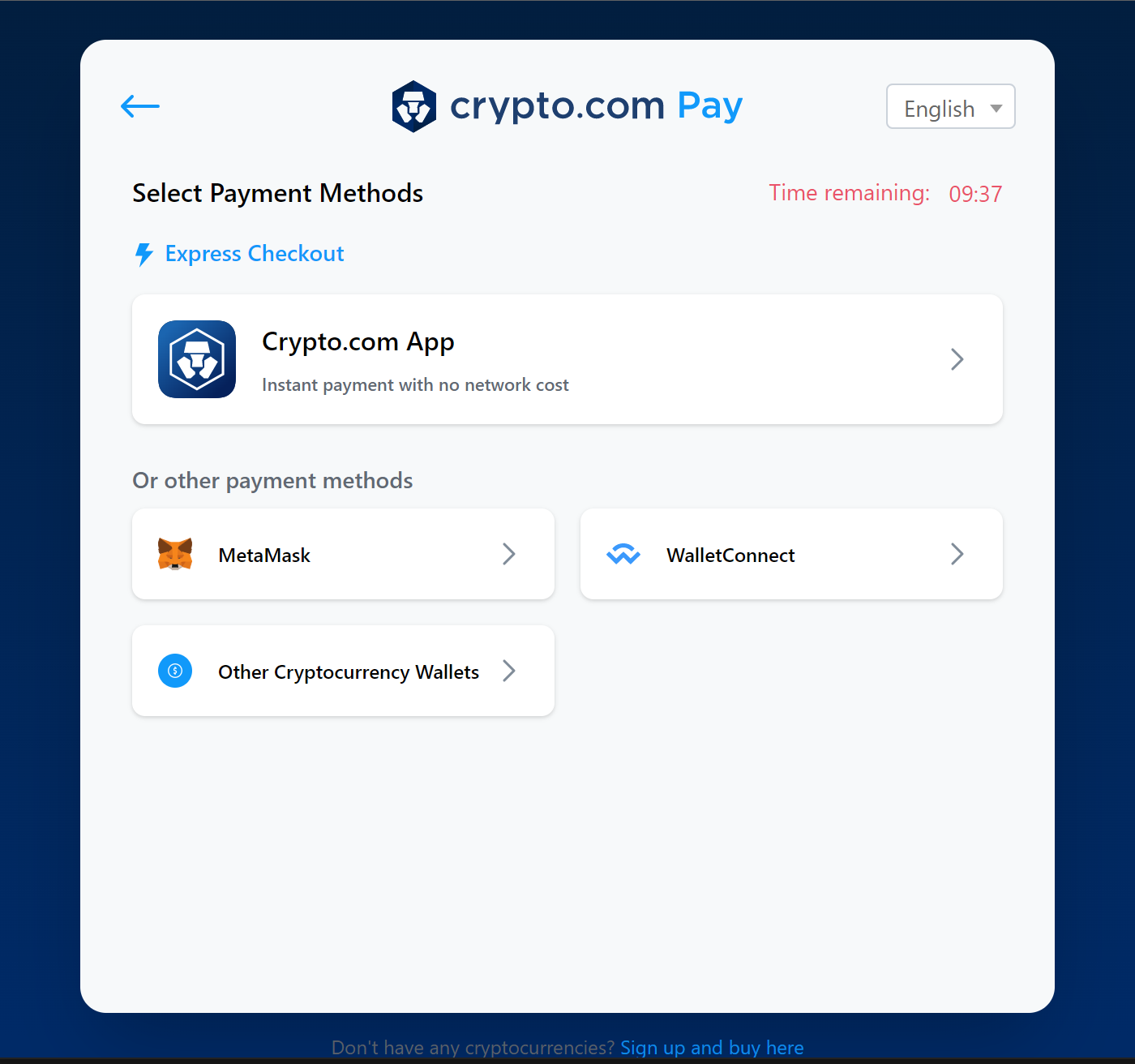The homepage for the crypto company is split into distinctive color segments. The top half and midway down the left and right sides feature a dark blue background. The bottom half, extending left and right until about half an inch from the bottom, transitions to a lighter blue, bordered by a black line.

In the top left corner, a blue arrow points to the left, adjacent to a six-sided polygon. Next to the polygon, there's a line outline and the face of a white block. To the right of this setup, "crypto.com" is prominently written in dark blue, followed by the light blue word "pay".

On the right side, there's a white tab labeled "English". Beneath the blue arrow, in black text, it says "Select Payment Methods". To the right of this text, the remaining time "9:37" is displayed in red.

Below this, another line reads "Express Checkout" next to a blue lightning bolt. There is a white tab spanning the width of the section, featuring the company's emblem on the left and the text "crypto.com app" to its right. Below, it declares "Instant payment with no network cost", followed by a greater-than symbol ">". The next line, in gray, reads "Or other payment methods".

Further down, three tabs are aligned, each going about halfway across the page. The first tab features a fox icon next to the text "MetaMask". The second tab has a blue 'W' with an arc above it, labeled "WalletConnect". The bottom tab contains a blue circle with a white border and an exclamation point inside, labeled "Other currency wallets".

At the bottom, right above the black border, small text reads: "Do not have any currencies? Sign up and buy here."